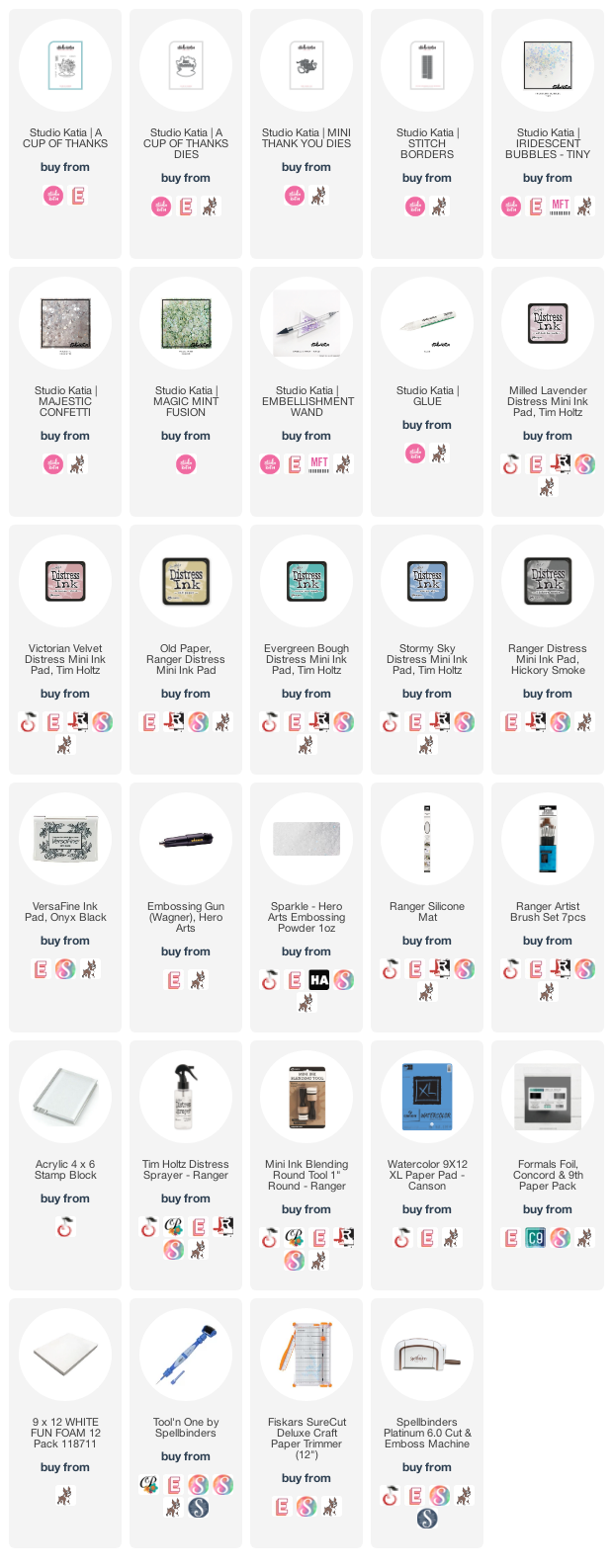The webpage features a grid layout consisting of five columns and six rows, organized into uniformly-sized boxes. Each of the boxes follows a consistent template. The first five rows are fully populated with five boxes each, while the sixth row contains only four boxes.

Within each box:
- A white circle at the top showcases an image of the product.
- Directly below the product image is a descriptive text that spans two to three lines, detailing the product.
- Following the description, there's a prompt that reads "Buy from," indicating options for purchasing.
- Beneath this prompt, there are one to five icons representing various purchasing platforms, differing in number depending on the product.

Overall, while each box maintains a similar structure, the featured products within the white circles are unique to each box.